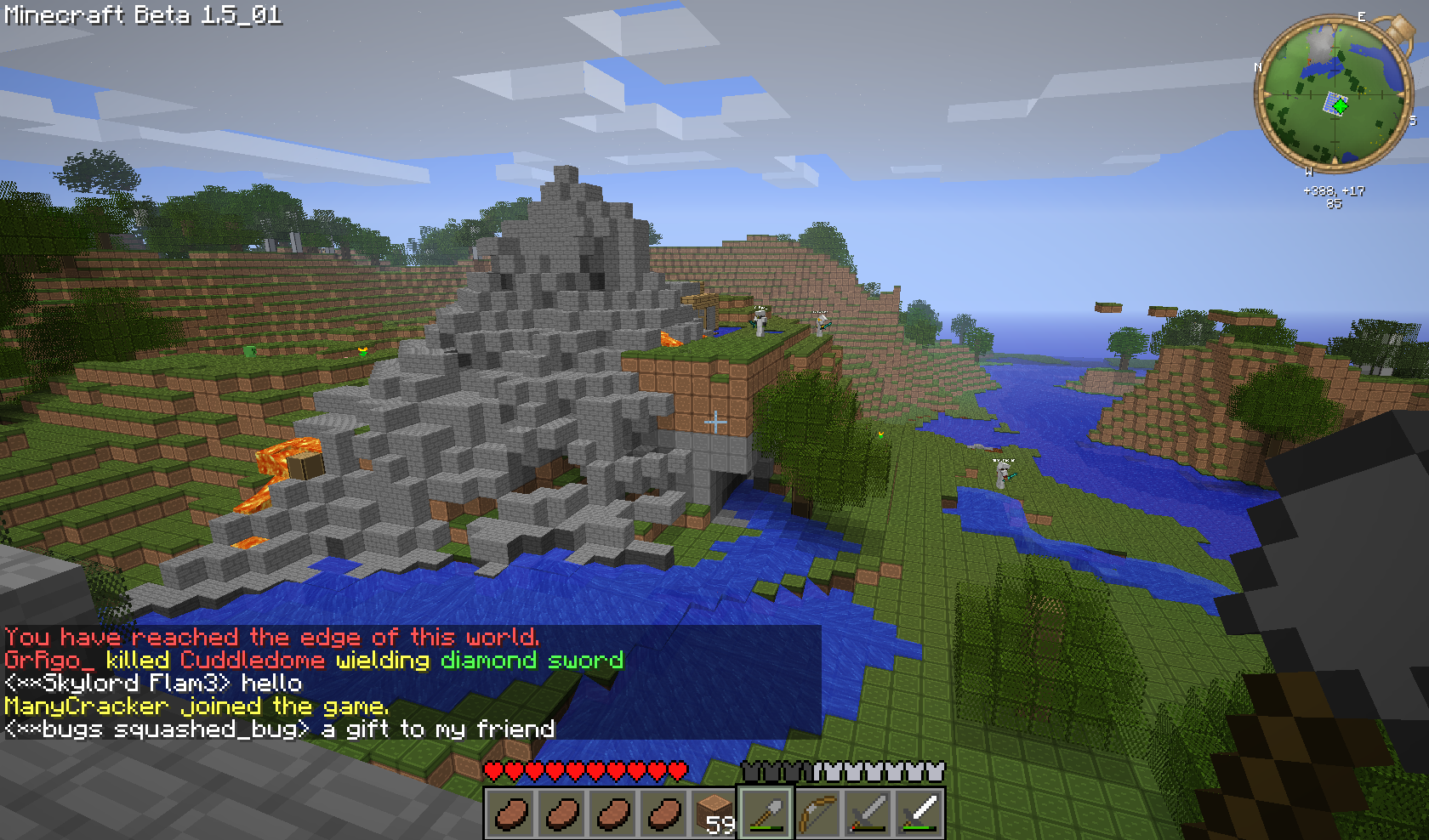This is a screenshot from the video game Minecraft, specifically from the Minecraft Beta 1.5_01 version, as indicated in white text in the upper left corner. The image captures a Minecraft world featuring a prominent grey mountain area surrounded by green grassy patches and multiple bodies of water. In the foreground, there's a noteworthy event message displayed in a large, transparent rectangle at the bottom left, which reads, "You have reached the edge of this world. GRRGO killed Cuddledome wielding diamond sword." The player’s status, including their remaining hearts and inventory, is also visible. On the right side of the image is a brown hillside area with another body of water. Notably, there's a circular map in the top right corner displaying various land features, such as green lands and darker green circles representing trees, along with blue areas indicating water bodies. The player appears to be holding a tool characterized by a gray metal tip on a wooden stick.